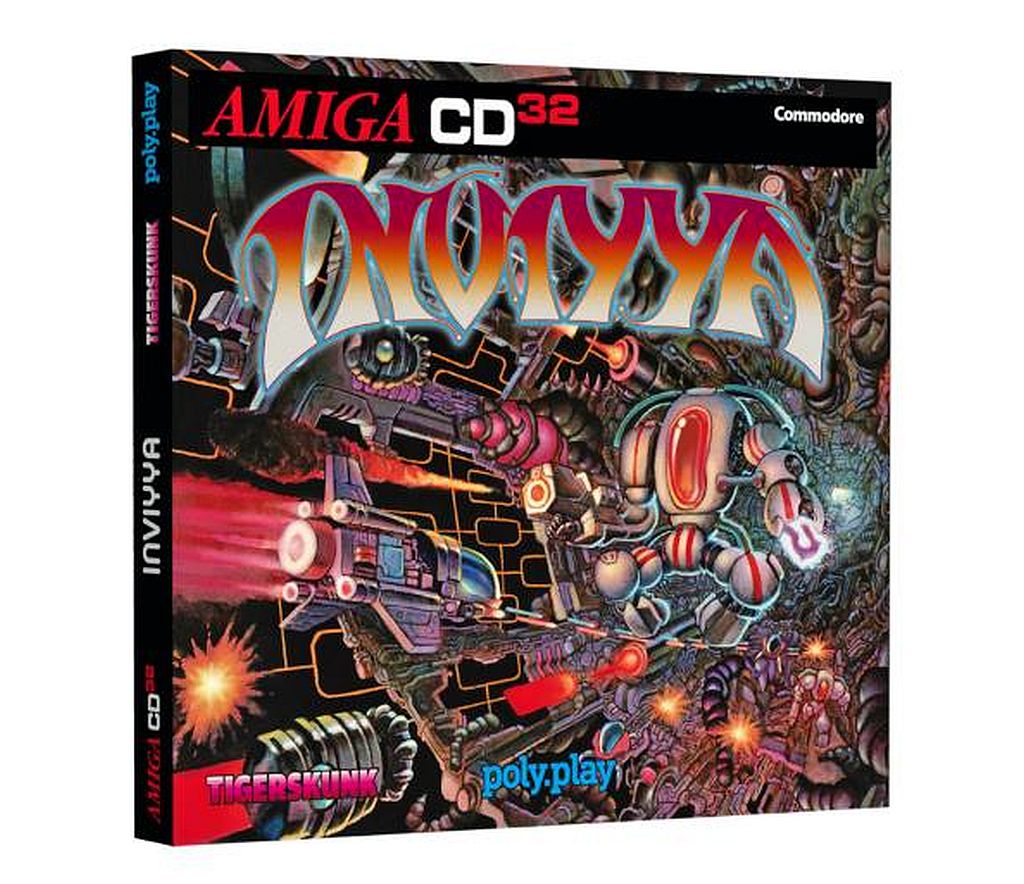The cover of this Amiga CD32 game "Inviya" is a striking and busy space-themed scene. The top section features a black band with "Amiga CD 32" in red and white text, alongside "Commodore" in smaller white text on the right. The main visual comprises a chaotic and detailed futuristic landscape, with rockets and intricate structures. On the left side, a rocket with flames shooting out trails into a scene filled with complex metallic lattices and various white and red robotic elements. The colorful and energetic background includes black space and an orange explosion. Centered across the top third of the image, the product name "Inviya" appears in large, bubble-style graffiti text, transitioning from a red band at the top through orange to a pale yellow at the bottom. The names "Tiger Skunk" and "Poly.play" also appear in pink and blue text, respectively, around the bottom of the cover. The CD spine, slightly tilted to the right, repeats the "Amiga CD 32" and "Inviya" branding, emphasizing its distinctive and retro video game appeal.